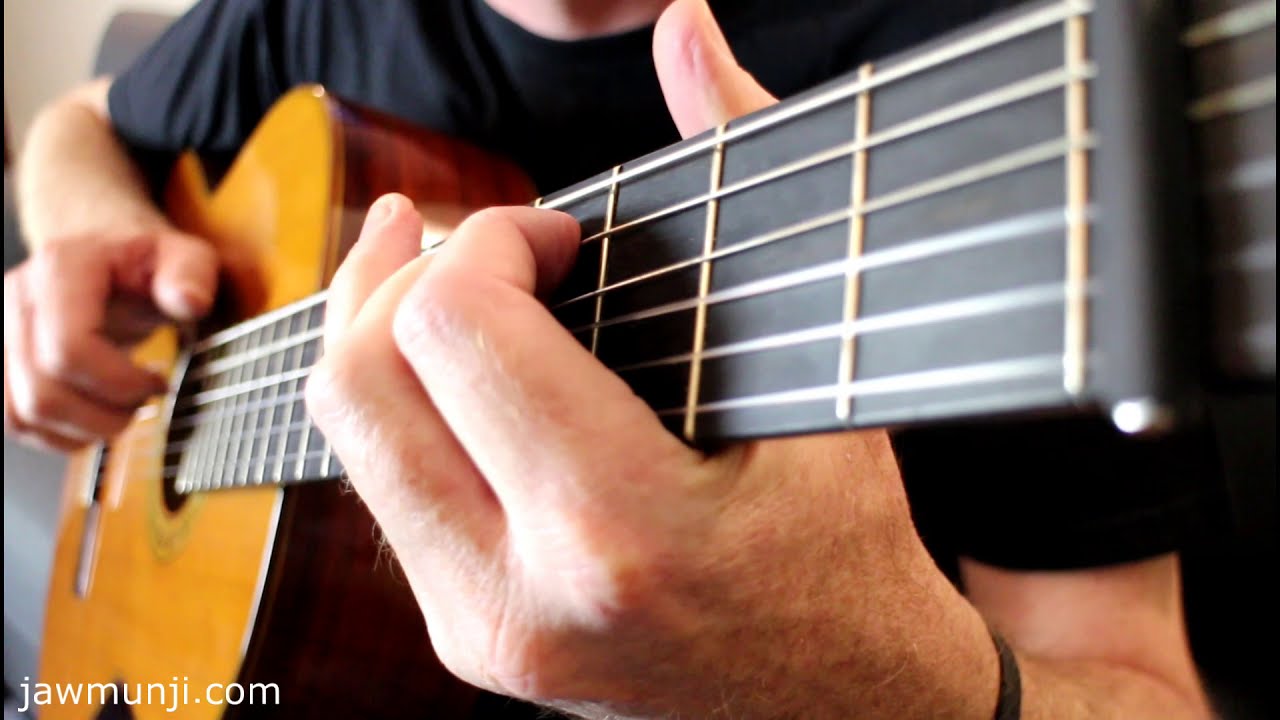The image is a close-up photograph of a man playing an acoustic guitar. The focus is on his hands, with his left hand forming a chord on the guitar's neck and his right hand strumming the strings near the base. The head and face of the man are cut off by the frame, leaving only a view from his neck downwards. He is wearing a black or dark blue t-shirt and a black bracelet on his left wrist. The guitar has a light yellowish-brown front with a dark hardwood, possibly walnut, wraparound on its sides. The neck of the guitar is black with gold bands. The text "jaamunji.com" appears in white lettering at the bottom left of the image. The overall composition features a clear focus on the hands and guitar neck, with the background becoming blurry towards the bottom of the frame.